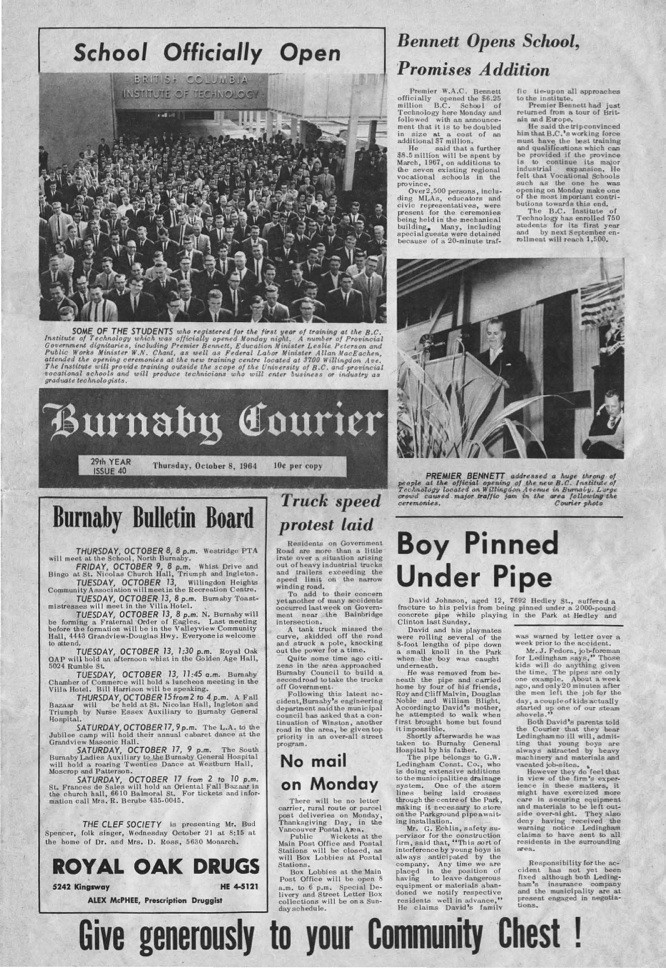The image depicts a greyscale newspaper page featuring multiple articles and photographs. The primary focal point is an article in the top left corner titled "School Officially Open," accompanied by a photograph of several people in coats and ties in a building marked as the British Columbia Institute of Technology. Directly below this, a text box with a black background and white font reads: "Burnaby Courier. 29th year, issue 40. Thursday, October 8, 1964, 10 cents per copy." Adjacent to the main article, on the top right, is another headline, "Bennett Opens School Promises Edition," with a photograph of a man speaking at a podium. Additional articles populate the lower section of the page, including a news story about a "Truck Speed Protest Lead," a notice of "No Mail on Monday," and a headline about a "Boy Pinned Under Pipe." Also visible is a community announcement, "Give Generously to Your Community Chest."